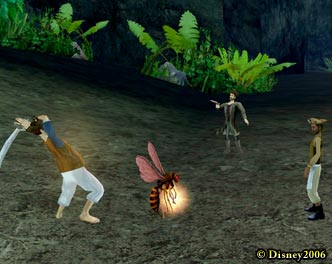This screenshot from what appears to be a Disney game, potentially the Pirates of the Caribbean MMO, captures a tense nighttime scene set in a tropical jungle. It features four characters and a large flying wasp. Along the top edge of the very dark background, there's a sparse line of large palm leaves erupting from the ground, hinting at the lush, exotic environment. At the center of the image, a man dressed in black with charcoal gray boots and a white shirt wields a gun in his right hand, aiming towards the bottom left corner. To his left stands another character in tan shirt and mid-calf brown pants, raising a sword overhead, ready to strike. In between these two characters is a gigantic wasp with glowing yellow light and reddish-brown wings. On the far right, another pirate-like character wearing a vest, white pants, dark boots, and a tri-point hat is visible, adding to the swashbuckling atmosphere. The hillside they stand on is brown and green, with ferns and other backlit foliage adding to the dimly lit jungle setting. The bottom right corner of the image bears a gold copyright mark that reads "Disney 2006".